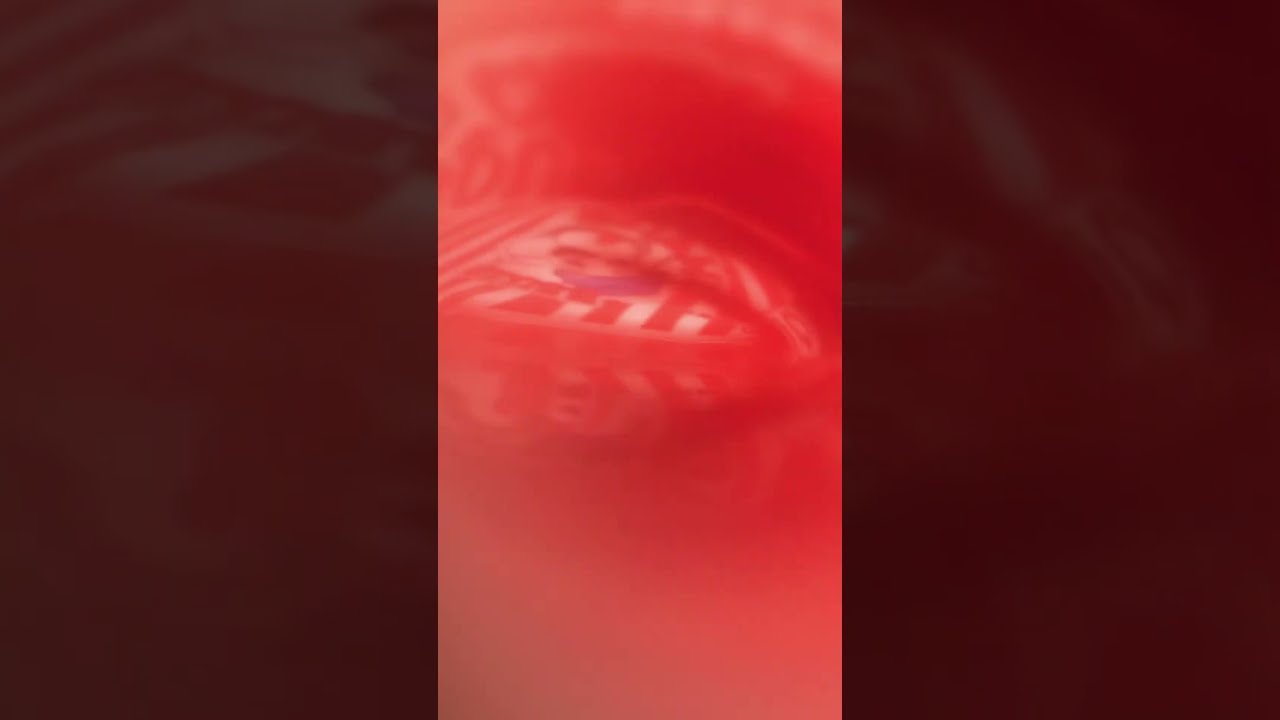This digital artwork presents a surreal and abstract depiction of an eye, dominated by a striking red color scheme. Central to the image is a stylized, somewhat distorted eye, in which the iris is a fuzzy, faint blue. The eyelid or surrounding area is patterned with white and red stripes reminiscent of a peppermint pinwheel. The artwork is elongated and rectangular in shape, with the main image centrally focused. The background consists of a darker red, blurred repetition of the central eye, adding to the image's disorienting and eerie ambiance. This piece, devoid of any text, blends elements of abstract art with an almost monstrous aesthetic, resulting in a captivating yet unsettling visual experience.